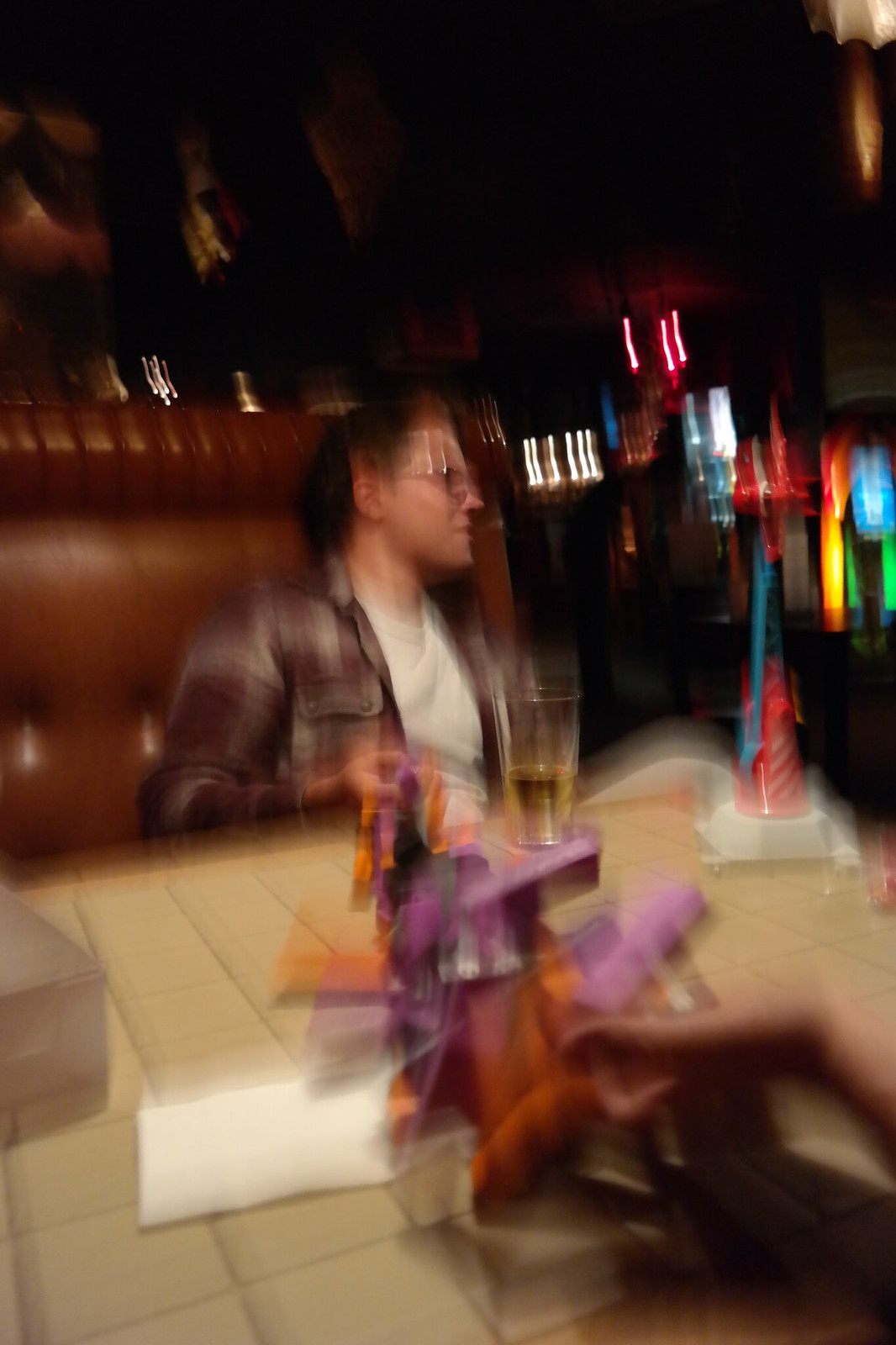This is a blurry photograph taken indoors at a restaurant, possibly capturing a celebratory moment, as a party hat can be seen to the right of the table. The image centers on a person with glasses, wearing a brown and white checkered shirt over a white t-shirt, and a necklace. They are seated in a booth with puffy brown leather seats that have a border around them. The table has a distinctive cream-colored square tile pattern. The person has a glass of beer in front of them, with about a quarter of the beer still left. They are sitting across from someone who is holding a purple and orange object. In the background, there are various colored lights—yellow, red, white, blue, and green—indicating a lively, party-like atmosphere. A napkin is also visible on the table. The image has a sense of motion and distortion, suggesting it was taken hurriedly or while the camera was in motion.